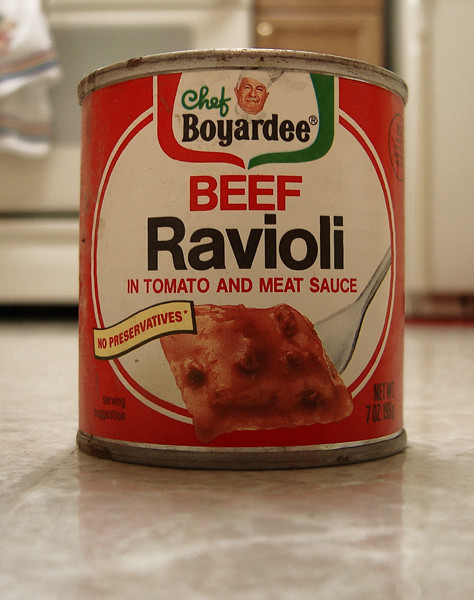The image showcases an old can of Chef Boyardee beef ravioli, prominently featured on a polished tile floor likely within a kitchen. The can, which appears significantly aged due to rust around the top metal edge, has a predominantly red label. At the center of the label, a white circle contains the green and black Chef Boyardee logo featuring a chef's face, with the words "Chef Boyardee" in green and black text respectively. Below the logo, "beef" is displayed in red text, followed by "ravioli" in large black letters, and "in tomato and meat sauce" written in red. The can also features a highly detailed close-up image of beef ravioli covered in sauce. A yellow ribbon to the left with red text declares "no preservatives," while the bottom right indicates "net weight: 7 ounces (199 grams)" and includes a "serving suggestion." In the background, various kitchen elements such as a white oven, a cabinet, and part of a refrigerator are visible, confirming the kitchen setting.